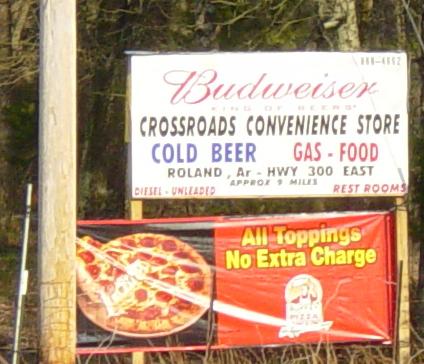This color photograph, taken outdoors during the daytime, features two prominently displayed signs attached to a single pole, with a lush backdrop of trees and grass. The upper sign, predominantly white with striking red cursive text reading "Budweiser," advertises the Crossroads Convenience Store. Below the Budweiser logo, bold black text informs viewers of cold beer, gas, food, and amenities available at Roland, Arkansas, Highway 300 East, approximately nine miles away. Essential services such as diesel, unleaded fuel, and restrooms are highlighted in red text on either side of the sign.

Directly beneath this main sign is a vibrant red banner advertising pizza. The banner showcases a tempting image of a whole pepperoni pizza, with one slice being lifted to display the stretch of melted cheese. In bright yellow text, the slogan "All toppings, no extra charge" is prominently featured. This visually appealing advertisement, combined with the informative convenience store sign, creates an inviting and attractive display against the natural greenery in the background.